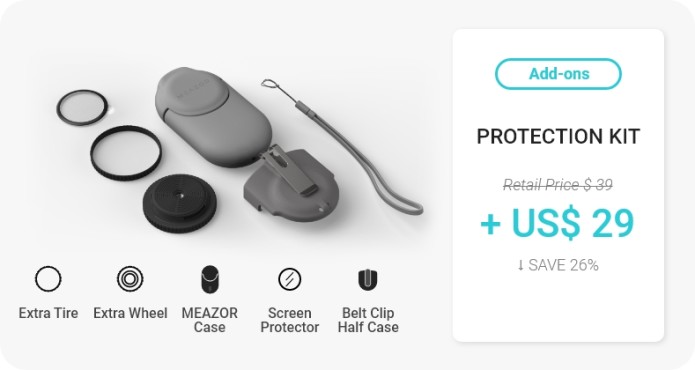The image appears to be a product listing, likely displayed on a website or mobile device, set against a very light gray background. To the right, there is a vertical rectangular box containing detailed information about available add-ons. The oval-shaped teal section at the top reads "Add-Ons." Below that, in large capital letters, it states "Protection Kit."

Following this title, the original retail price of "$39" is shown in gray and crossed out. Beneath the crossed-out price, a bold teal font highlights the new price as "$29", noting a 26% savings.

To the left of this box, the image showcases five items included in the Protection Kit: an extra tire, an extra wheel, a measuring case, a screen protector, and a belt clip half-case. Above these descriptions, the images of the items are displayed. The first three items on the right are circular: two are transparent, and the third is solid black. Adjacent to them is a gray piece, which seems to be attached to another element, and a gray clip, indicated as the belt clip.

This image provides a comprehensive overview of the Protection Kit, detailing both the components and the updated pricing in a clear and organized manner.